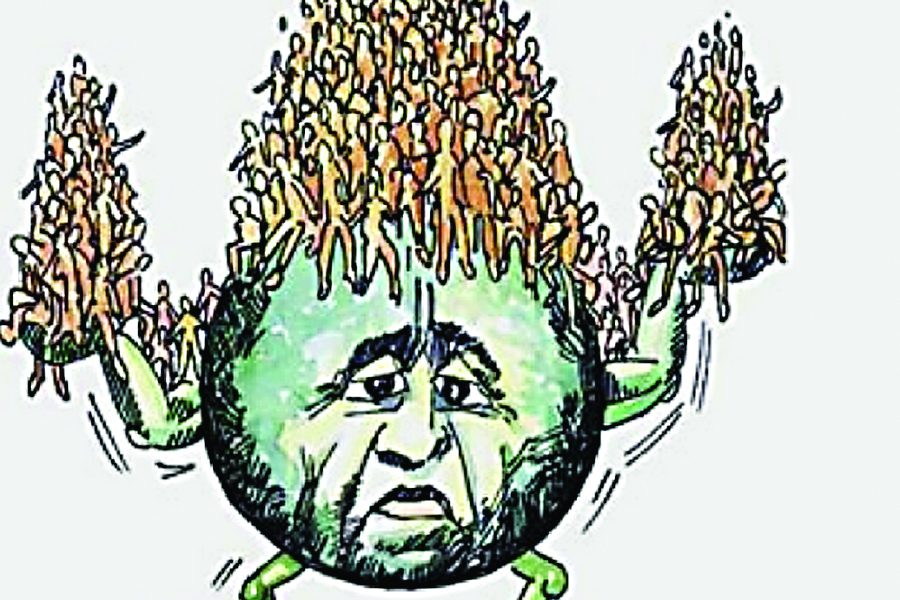This detailed cartoon image portrays a green, spherical figure resembling a lemon but with human features such as realistic eyes, a nose, a mouth, and expressive wrinkles and eyebrows. This figure, often interpreted as a personified Earth, appears burdened and weary, indicated by its frowning expression. The cartoon Earth stands on two skinny legs and extends its two green arms upwards, holding up masses of blank-faced figures. Each arm supports about 30 individuals, with an overwhelming number, ranging from 50 to 75, precariously stacked on its head. Motion lines suggest the arms and legs are trembling under the strain, emphasizing the figure's struggle and the daunting weight of the human figures atop it. The backdrop is entirely white, bringing the central theme of burden and struggle into sharp focus.